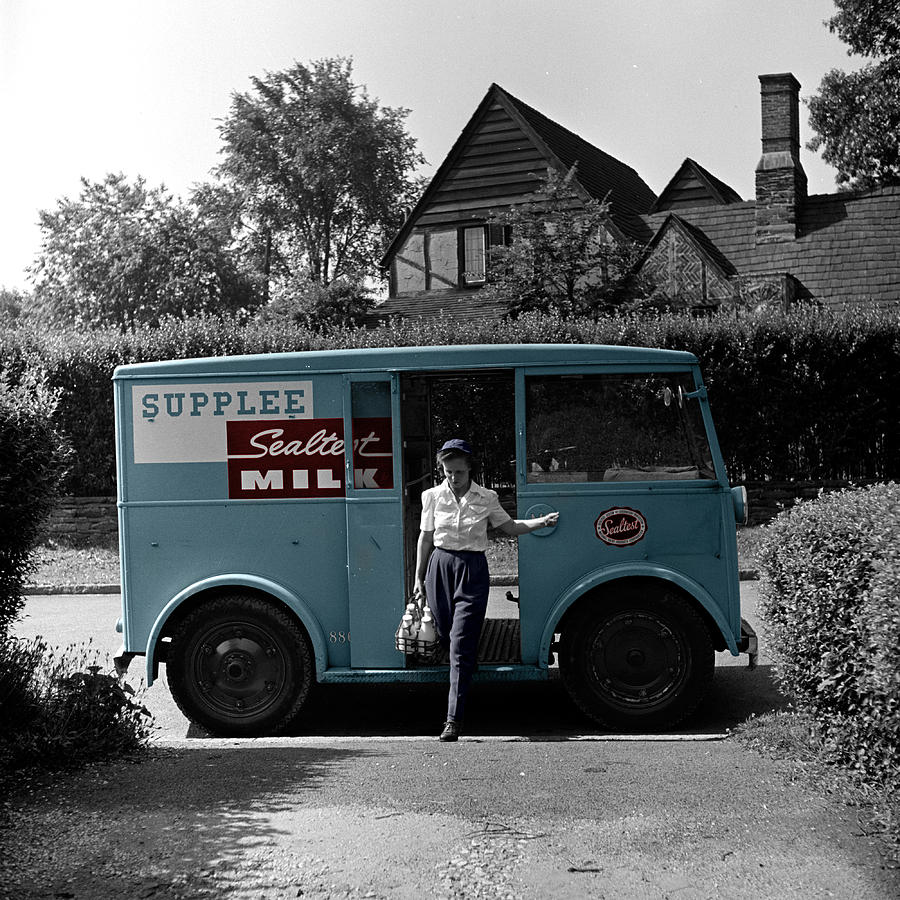This black-and-white photograph, likely from the 1950s or 60s, captures a milk delivery scene with nostalgic charm and striking detail. The image centers on a vintage aqua blue box truck labeled "Supply Sealtest Milk" adorned with a red oval seal reading "Sealtest" in white cursive. A milkwoman is captured stepping out of the truck, with one foot already on the driveway lined by bushes. She wears a neatly pressed white short-sleeved button-down shirt, high-waisted blue slacks that taper at the ankle, and a matching blue hat. She carries a sturdy metal crate filled with glass milk bottles. The background features a house with a triangular roof and chimney, partially obscured by thick bushes and surrounded by trees. The scene, emphasizing the quintessential mid-20th-century milk delivery service, provides a charming glimpse into a bygone era.